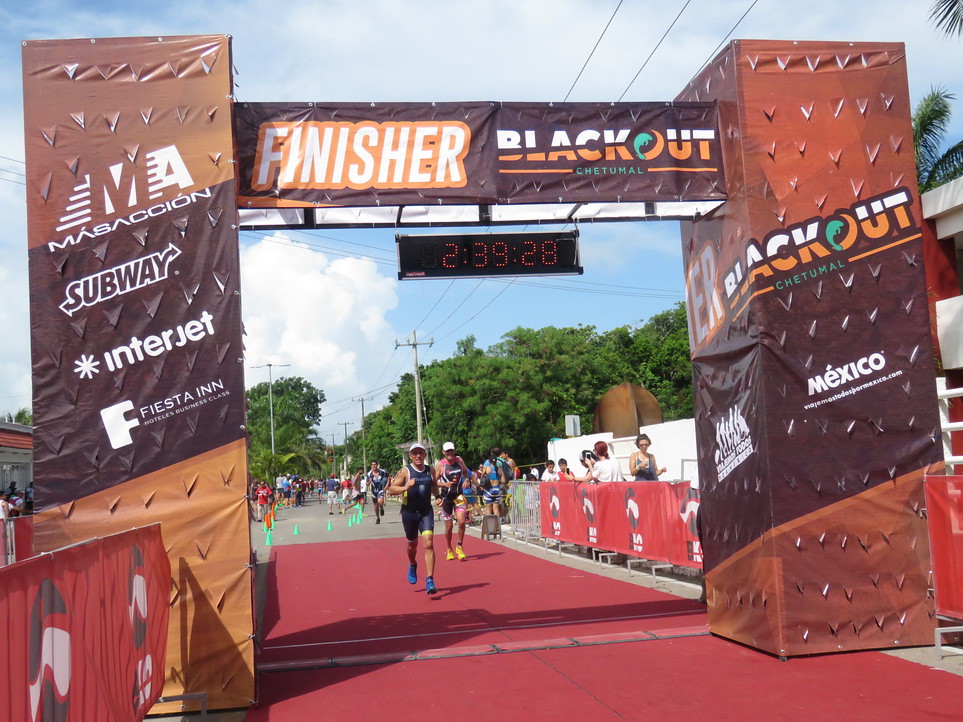The photograph captures the dramatic finish line of a marathon, signified by a large gateway with the words "Finisher" and "Blackout" prominently displayed on top, and "CHETUMAL" in smaller letters beneath. A digital timer hanging from the center of the gate shows 2 hours, 39 minutes, and 28 seconds. The gateway structure features dark colors, mainly red, brown, and black, and decorative columns with triangular cutouts, adorned with sponsor logos including MASACCION, Subway, Interjet, and Fiesta Inn.

In the forefront, two middle-aged to older male runners are sprinting towards the finish line. The runner in the lead is wearing a white cap, a black tank top, black shorts, and blue shoes. Trailing closely, the second runner sports a white baseball cap, a tank top with red edges, reddish-black shorts, and yellow shoes. They are both running on a red concrete surface marked by green cones that direct the runners' path. 

Beyond the gateway, spectators stand behind barriers, eagerly cheering the runners on. The background is lined with trees and telephone poles, adding a natural and urban mix to the scene. The energy and enthusiasm of both participants and supporters are palpable, capturing the spirit of the race.